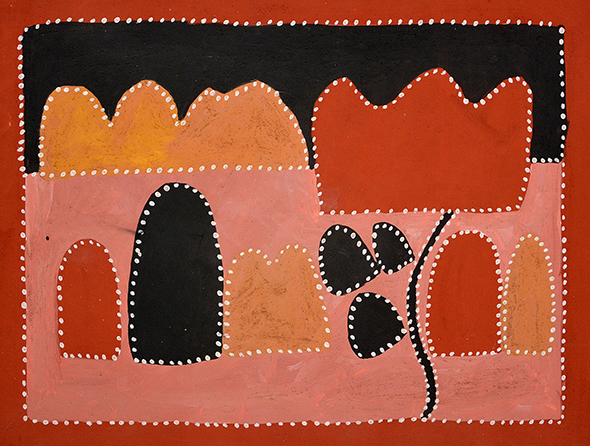This modern abstract painting features a sophisticated use of four primary colors: copper, black, pink, and bronze. The composition is horizontally oriented and rectangular, with a border defined by white dots and a broader bronze outline. Within the pink background of the lower two-thirds, several doorway-shaped patches adorned with white dots are visible. These patches come in red, black, and tan, each resembling small pockets or crowns. On the left, there's a red patch shaped like a door, followed by a larger black patch, then a tan, M-shaped object, all surrounded by more white dots. Towards the right, three smaller black objects, flanked by red and tan patches, all share the white-dotted motif.

In the upper third, the background shifts to black, featuring two crown-like shapes, one tan and one red, each outlined by white dots. To top off the intricate detailing, a black swirling line navigates from beneath the crown shape, extending to the bottom edge of the painting. The piece emanates a floral and plant-like abstraction, invoking imagery of a rose with its stem, all encased in a richly dotted texture, emphasizing its modern artistic flair.